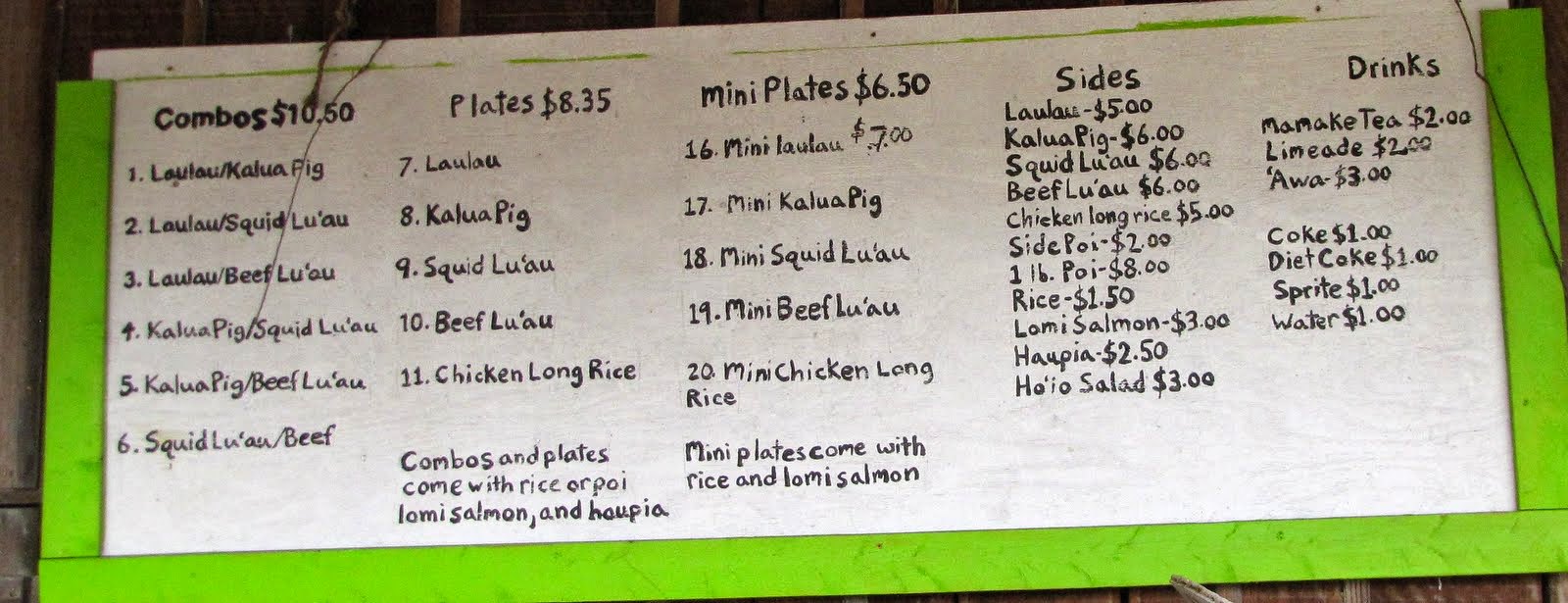The photograph captures a neatly organized, landscape-oriented menu on a long white piece of paper. The menu is bordered by a vibrant green background, creating a striking contrast. In the top left corner, the menu advertises "Combos for $10.50" in bold lettering. The menu is meticulously handwritten in black ink, listing a variety of food options under different headings.

On the left side, there are "Plates" priced at $8.35, featuring items such as squid and beef. Adjacent to this, the "Mini Plates" section offers selections for $6.50, with choices including squid, beef, and mini chicken long rice.

To the right, a column dedicated to sides lists options ranging from $3.00 to $6.00. Further to the right, a drinks column displays beverages like limeade for $2.00, IY for $3.00, and both Coke and Diet Coke for $1.00 each.

The menu, though simple, is clearly structured to offer a range of options, emphasizing both the variety and affordability of the offerings.